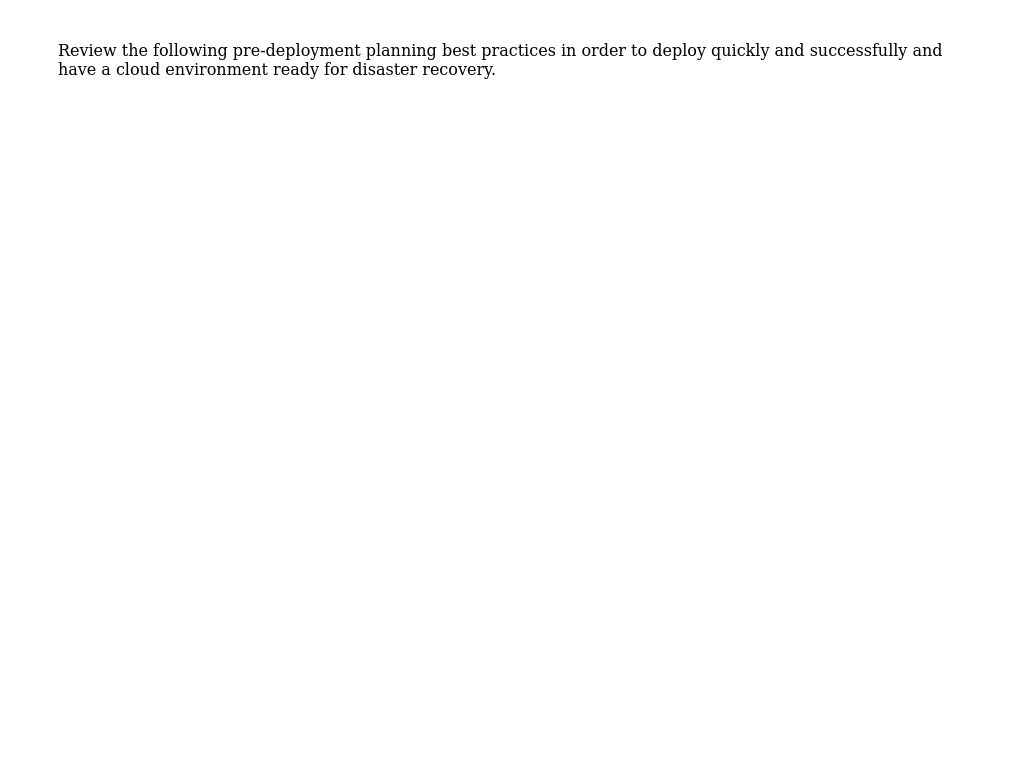The image features a stark white background with a single line of black text centrally positioned at the top. The text reads: "Review the following pre-deployment planning best practices in order to deploy quickly and successfully and have a cloud environment ready for disaster recovery." This minimalistic presentation, devoid of any additional graphics, logos, or identifiable platform elements, makes it unclear whether the image originates from a website, application, or digital device such as a phone or PC. The content appears to target professionals involved in software or web application development, emphasizing the importance of thorough pre-deployment planning for efficient deployment and disaster preparedness. The simplicity of the visual suggests that the actual best practices might be detailed on a subsequent, unseen page.